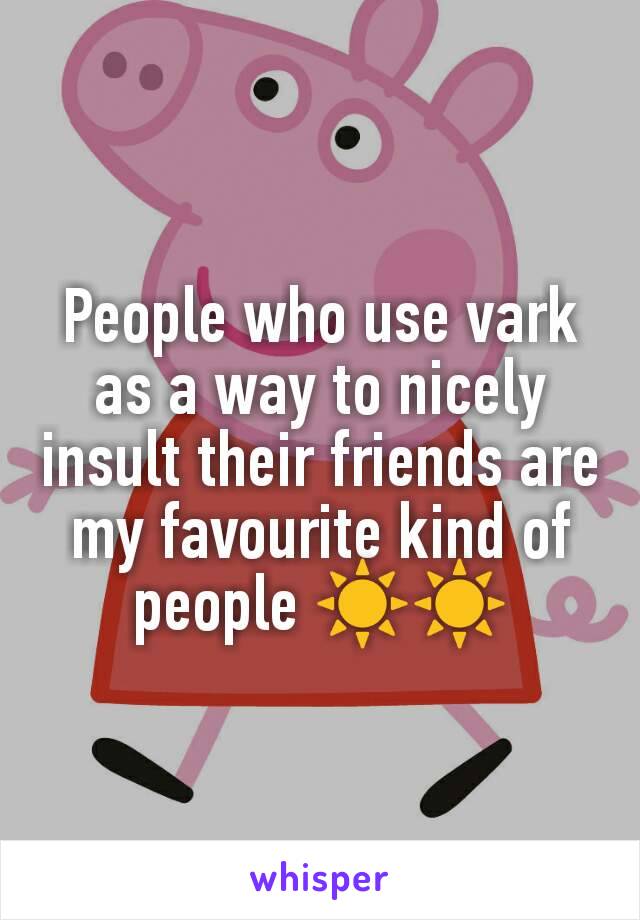This detailed illustration features the cartoon character Peppa Pig against a gray background. Peppa Pig is depicted as a simple, pink cartoon pig with a round head, an extended snout with two black nostrils, two oval-shaped ears, two eyes with black pupils, and rosy pink cheeks. She has a pink curly tail and wears a bright red dress with black shoes. Overlaid on the image, in large white text with a black drop shadow, is the quote: "People who use VARK as a way to nicely insult their friends are my favorite kind of people," flanked by two bright yellow sun emojis. Additionally, at the bottom of the image, there is small text in a purple font that reads "Whisper."